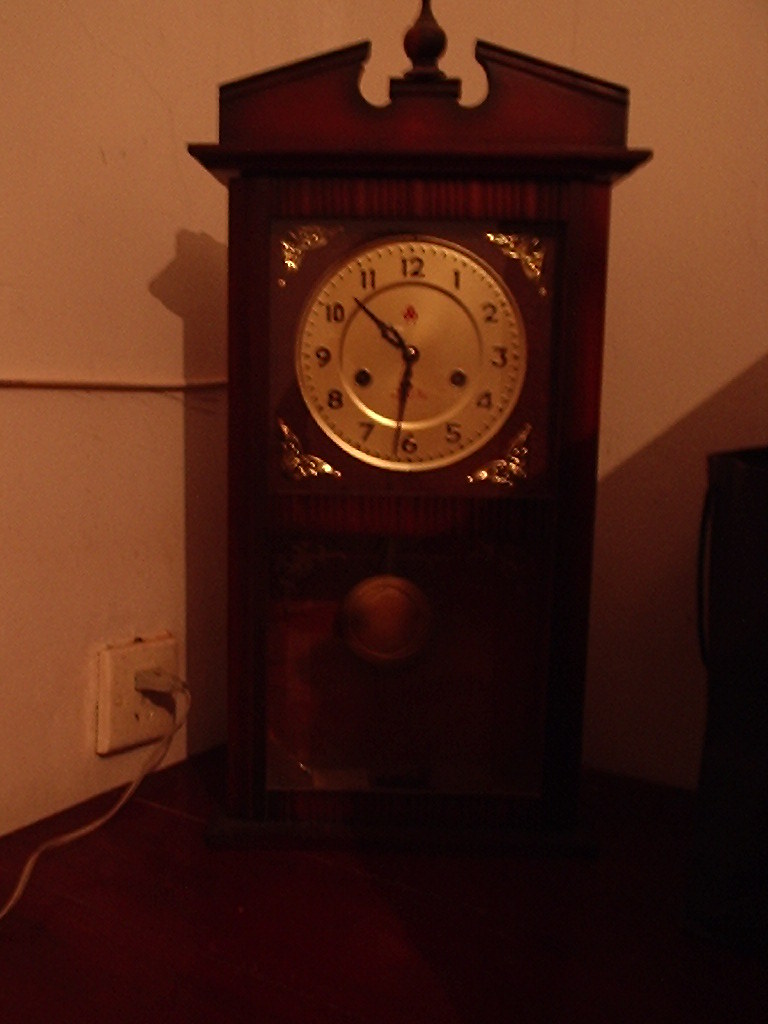This photograph showcases a vintage, table-top clock, elegantly positioned on a dark wooden surface. The clock features a smaller, square face encased in a rectangular frame. A distinguishing characteristic is its brass or metal pendulum visible at the bottom. The clock face itself is pristine white, adorned with numerals in a dark hue or possibly gold. These numerals are complemented by delicate golden splotches and decorative elements that adorn the corners. The clock's design is further enhanced by intricate carvings that culminate in a peaked top, complete with artistic cutouts. On the left side of the image, an older-style light gray cord is visible, indicating that the clock is electrically powered.